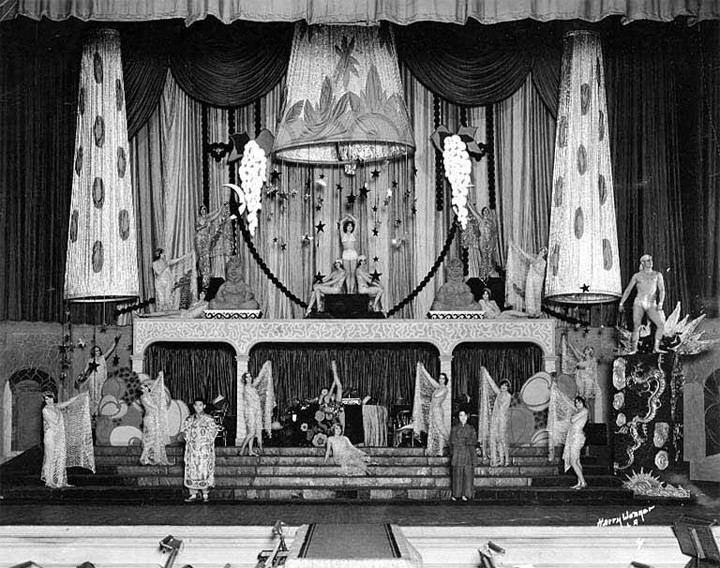In this black and white photograph, we see an elaborate, multi-level stage that appears to be from the 1920s. The stage, adorned with intricate curtains and drapery, features two levels stacked upon one another. At the very top, a raised curtain and side drapes with dark circular designs frame the scene. Dominating the center is a large, leaf-patterned lampshade in white and gray.

On the upper level of the stage, a woman stands prominently in a white bikini, her hands raised in a dramatic pose, drawing attention from the fellow performers surrounding her. Flanking her legs are two other scantily clad women, while various other figures across the stage, including a man in Speedo-like trunks, add to the tableau. Entranced, the ensemble casts their gazes and gestures towards the central figure.

Below, the stage extends downward to a series of steps occupied by numerous people in lace outfits, with their hands also lifted in the air, creating a dynamic and unified display. Towards the bottom right, a man stands on a column adorned with a striking light design. The base of the stage likely includes an orchestra pit, hinted at by the presence of musical equipment in the background. The image captures a moment of intricate, staged grandeur, reminiscent of early 20th-century theatrical performances or spectacular Las Vegas shows.